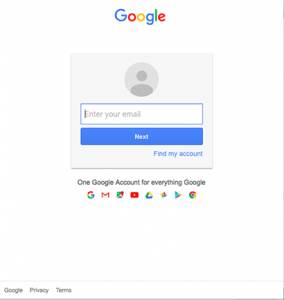The image features a clean interface characterized by several distinct visual elements. A grey line borders the bottom edge and the right-hand side of the image. Dominating the center is the prominent "Google" logo, showcasing the letters in a vibrant color scheme of blue, red, yellow, blue, green, and red. Below this, a grey square houses a darker grey circle, which contains an icon of a person.

Further down, a rectangle with a blue outline presents some text in grey. Below it, another blue rectangle contains a word, with additional blue text beneath it. The caption, "One Google account for everything Google," is clearly visible underneath these elements.

Various service icons are displayed beneath this message. These include the iconic Google and Gmail logos, alongside other less discernible symbols: a red rectangle with a white spot, a couple of indistinguishable icons, followed by a logo that seems to hint at Google's Chrome browser with blue and yellow hues.

At the bottom, there is another grey line followed by some white space, concluding with the words "Google," "Privacy," and "Theme" set apart by grey dividers.